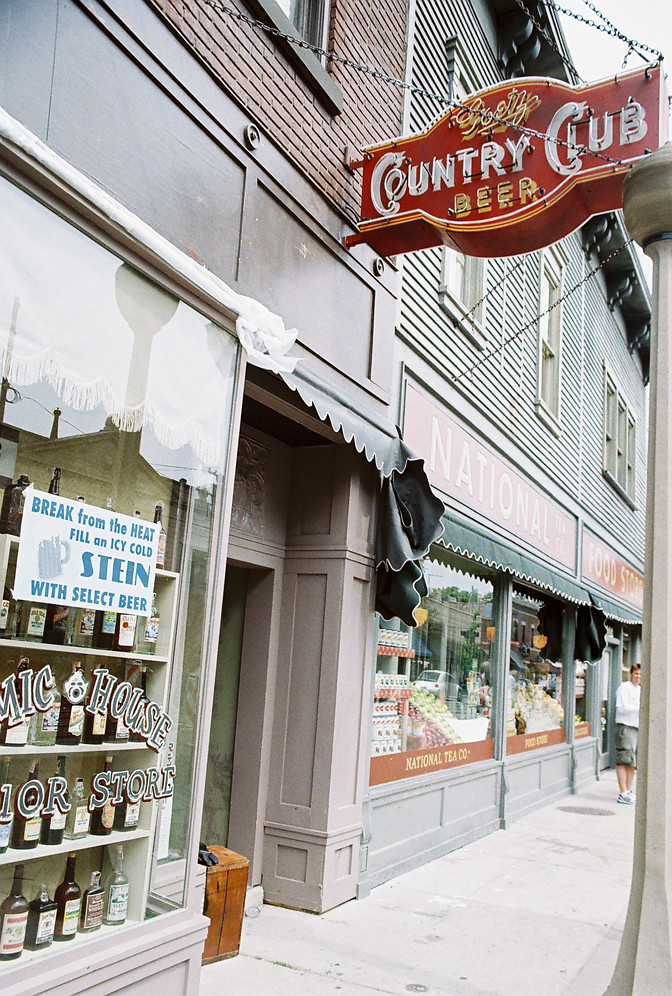The photograph captures a daytime scene of a sidewalk in a downtown area, possibly Nashville. The focal point is an outdoor storefront with a red, neon sign displaying the words "Country Club Beer" in white and yellow lettering. The sign is attached to the side of a gray and brown building with overhangs and awnings. Although the neon sign is not lit, it prominently marks the entrance of what appears to be a liquor store, evidenced by the visible liquor bottles through the large front windows. The sidewalk in front of the store is white, and the setting suggests a small town or city atmosphere. A single individual stands in the background on the far right, looking directly at the camera as the picture is taken at an angle.